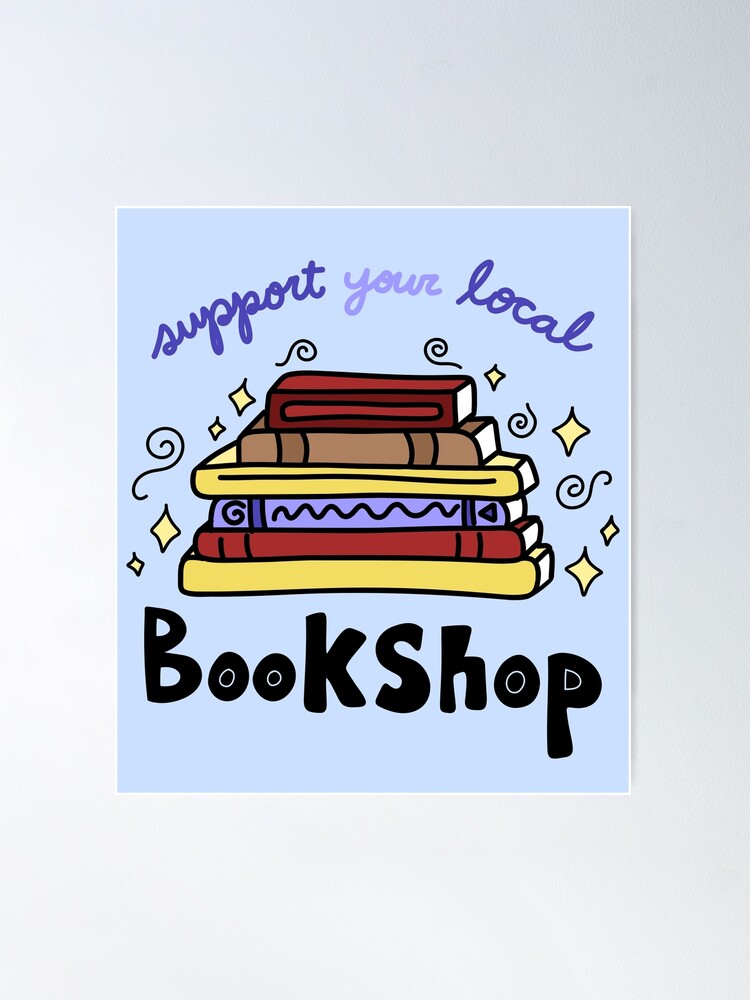The image is a colorful poster set against a plain gray background, depicting an artistic and eye-catching promotion for local bookstores. In the center, a blue card features the handwritten cursive message "support your local" in varying shades of purple, creating a gradient effect with "your" being lighter. Below this, in bold black letters with tiny white circles inside the O's, is the word "bookshop." The focal point of the poster is a stacked pile of six books, artistically illustrated with a whimsical touch. The books display a sequence of colors from top to bottom: red, brown, yellow, purple, red, and yellow, each surrounded by golden sparkles and dynamic whirly swooshes, suggesting movement. Additional decorative elements like diamond emblems, music clefs, and squares float around the stack of books, enhancing the lively and festive atmosphere of the design. This poster effectively encourages support for local bookstores amidst the challenges posed by the rise of e-books, aiming to reignite the excitement for reading.